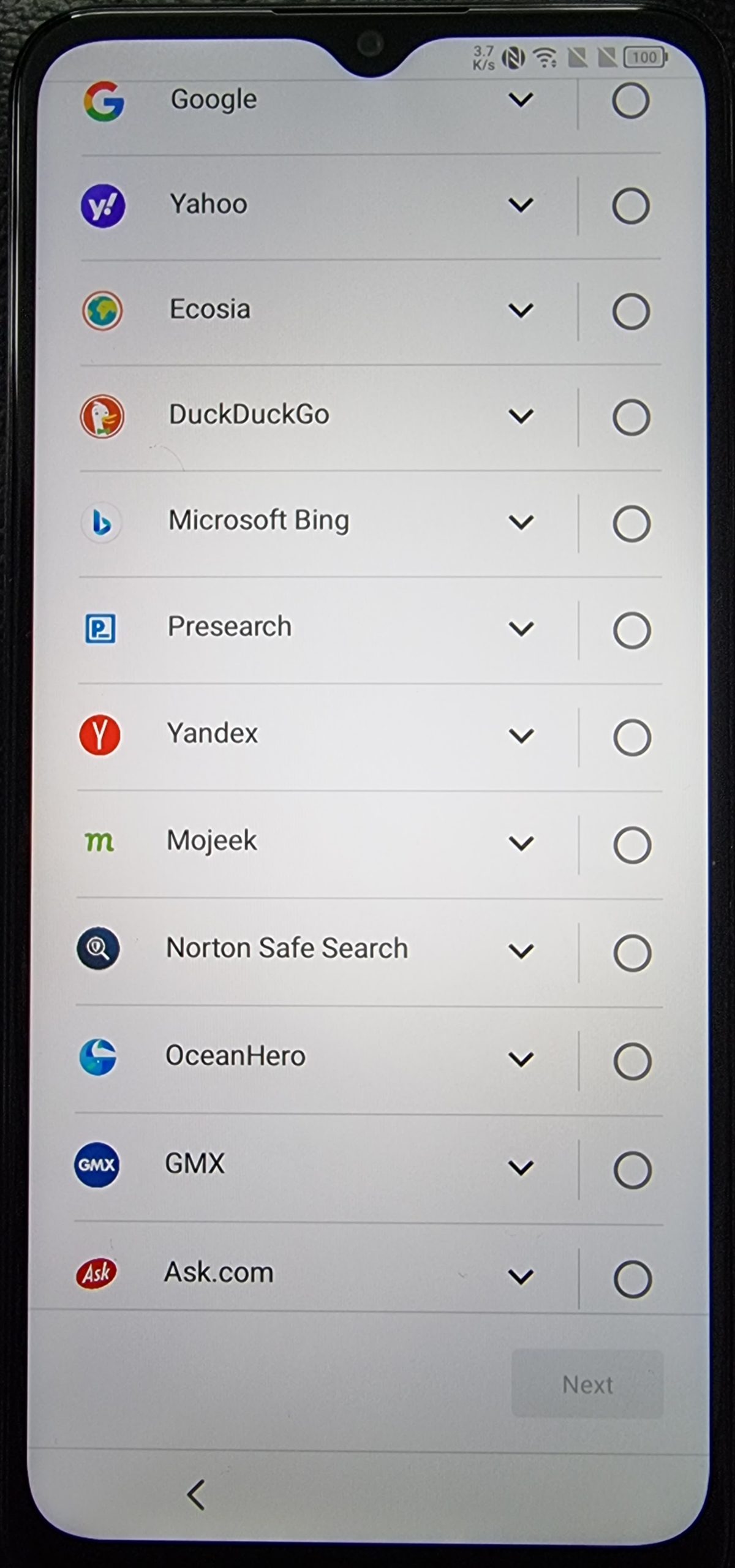A photograph captures the screen of a smartphone placed on a gray carpeted floor. The phone's battery is fully charged, indicated by the 100% icon in the upper left corner of the screen. The display shows a list of search engine apps arranged vertically. Each app is accompanied by its respective icon on the left side, followed by its name. To the right of each app's name, there is a downward-facing arrow button, and the far right side of each line displays a clickable circular icon. The apps listed from top to bottom are Google, Yahoo, Ecosia, DuckDuckGo, Microsoft Bing, Presearch, Yandex, Mojeek, Norton SafeSearch, OceanHero, GMX, and ask.com. At the bottom right of the screen, there is a light gray box with an option to click "Next."